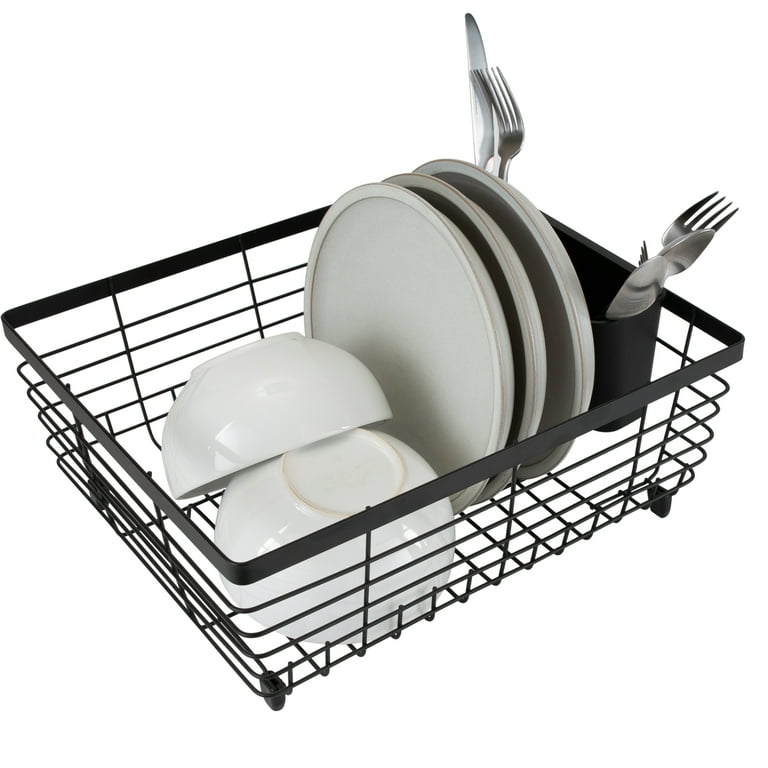This image is a detailed, color photograph in landscape orientation, featuring a black wire dish drainer set against a stark white background, giving the impression it is floating. The rectangular-shaped dish drainer is positioned at an angle, with its short sides facing the bottom left and top right corners of the frame. 

Inside the dish drainer, there are three large white plates standing upright near the top right section, while two large white soup bowls are placed on their sides in the lower left corner. The light reflecting off the bowls suggests that the original photo was taken in a well-lit environment, possibly with natural or kitchen lighting, before being edited onto the clean background.

Attached to the dish drainer on the top right is a black elliptical utensil holder. This holder contains silverware, specifically two stainless steel forks, two spoons on the right side, and a butter knife alongside a fork on the left side. The construction of the dish drainer and utensil holder is a black iron or steel metal grid, giving it a simple yet functional appearance.